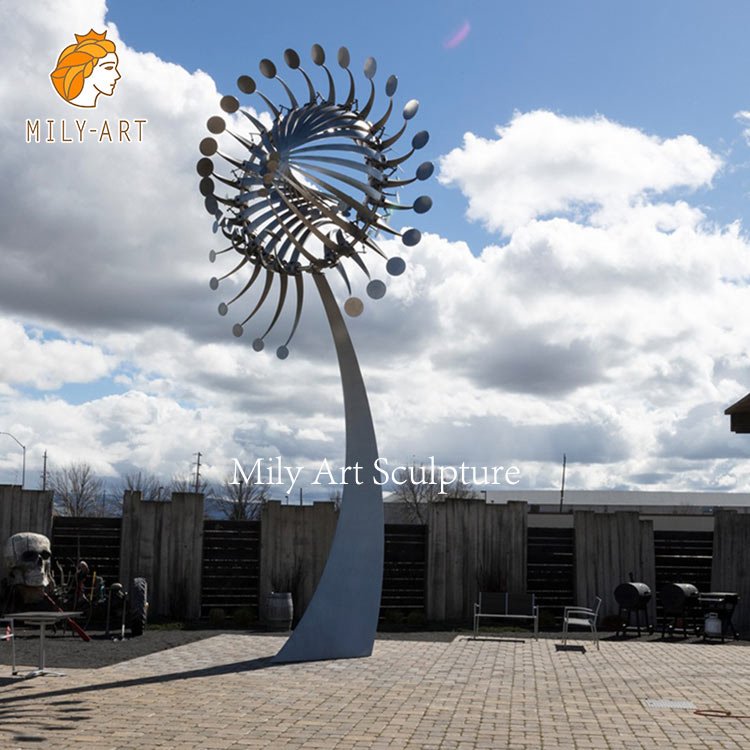In the image, we observe a tall, silver sculpture that prominently stands on a gray and reddish brick ground. This sculpture, identified as the "Miley Arts Sculpture," features a windmill-like structure at its peak, with blades resembling spoons arranged in a circular pattern.

On the far left side of the image, at the bottom, there is a significant gray skull situated next to a black tire. A table is positioned nearby the skull. The scene is bordered by a wooden fence featuring uneven lengths and a dark brown hue. Adjacent to the sculpture, on the right side, there are silver and brown benches, and further back, black grills are visible.

The backdrop includes a sky of clear blue, adorned with fluffy white clouds. In the upper left corner of the image, a depiction of a woman with blonde hair and a golden crown is noticeable, along with the text "Miley Arts." This detailed scene merges artistic elements with an assortment of everyday objects, creating a unique and intriguing visual composition.